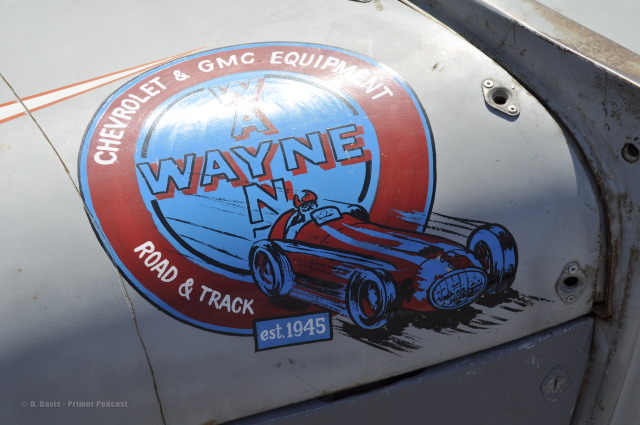The image shows a close-up of a sticker placed on a curved, possibly metallic, surface that appears to be part of a car or mechanical equipment. The surface is gray with some dirty, rust-colored spots on the right side. The sticker has a blue circular border with a red circle inside it. Within the red circle, in white letters, it says "Chevrolet and GMC Equipment." At the bottom of the sticker, there is a blue rectangle that reads "Established 1945." In the center of the sticker, there is an image of a vintage race car with a driver wearing a red helmet. The words "Road and Track" are also displayed on the sticker. Additionally, within a smaller blue circle at the very center, the word "Wayne" is written both horizontally and vertically, intersecting at the letter 'Y'.